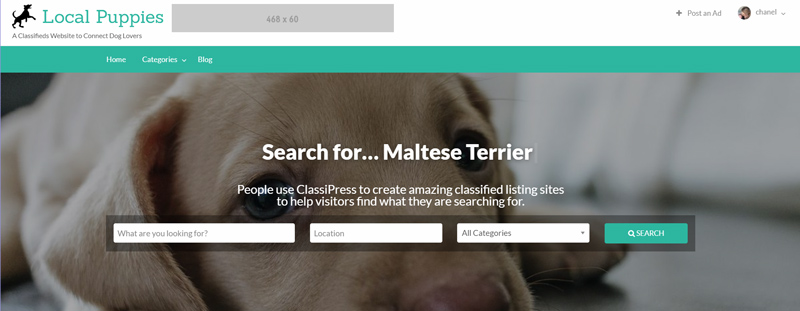The image is a rectangular banner with the long side extending horizontally. A white border outlines the top edge. In the upper left corner, a symbol of a black dog standing on two legs is accompanied by the green text "Local Puppies." Beneath this, in smaller font, it reads "Classified Websites to Connect the Lovers."

To the right of this is a gray box containing the text "4868 by 60." Further to the right, there is a plus symbol, the phrase "Post an ad," a circle with a sewing needle icon, and an unreadable word.

Below this top section, a green banner spans the entire width of the image. In white text, it lists "Home," "Categories," and "Blog." Below the banner, there is a picture of a tan puppy gazing to the right. Superimposed on this image in white writing is the phrase "Search for Maltese Terrier."

At the bottom of the image, it states, "People use ClassyPress to create amazing classified listing sites to help visitors find what they are searching for."